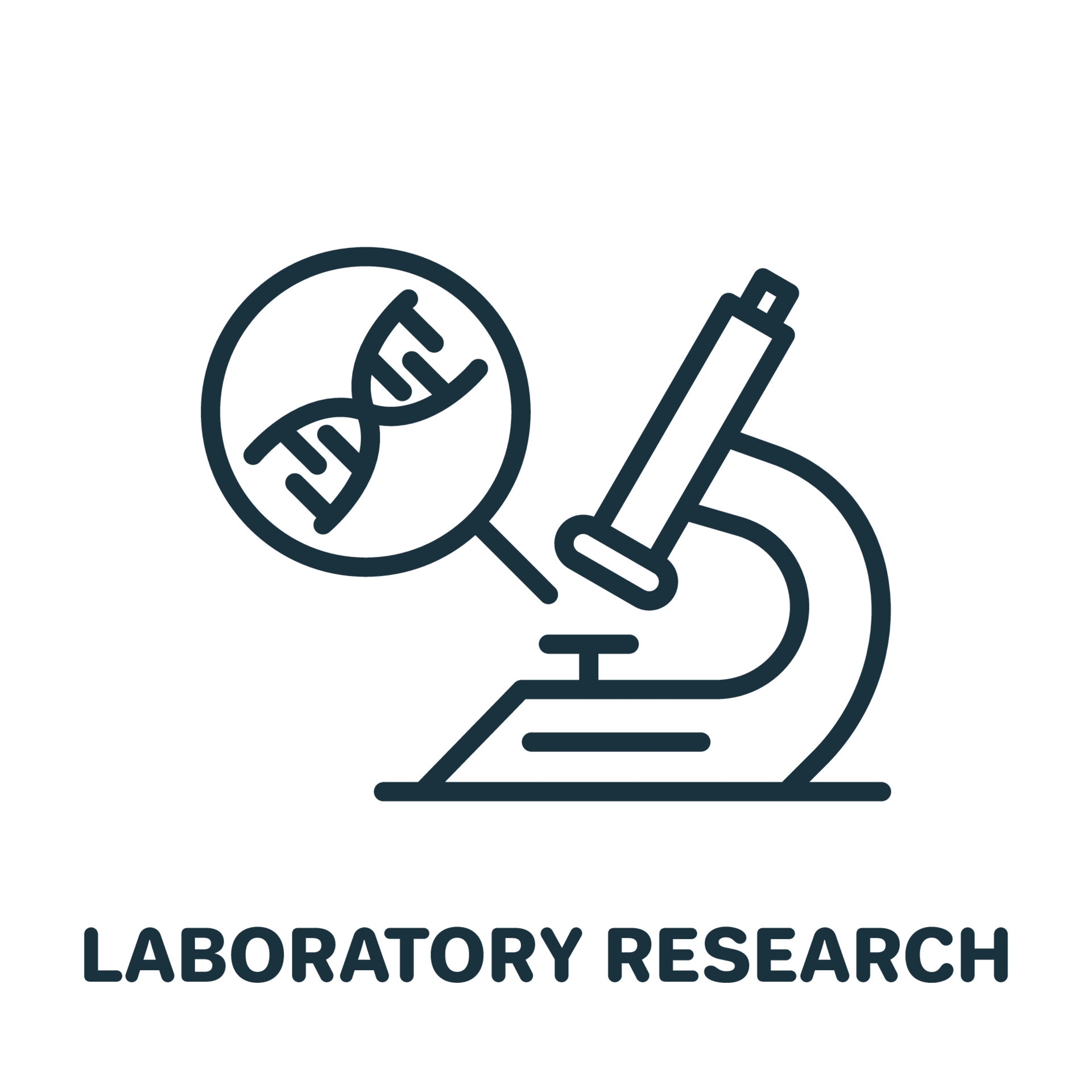The image is a graphical sign on a white background, predominantly featuring black elements. At the bottom, spanning nearly the entire width, the text "LABORATORY RESEARCH" is displayed in an all-caps, curved-edged font. Above this text, on the right side, there is a simplistic icon of a microscope. To the left of the microscope, a black line points upward into a circle located in the upper left portion of the image. Inside the circle, there is a depiction of a DNA helix. The entire design is minimalist, using only black lines and text to convey its message.